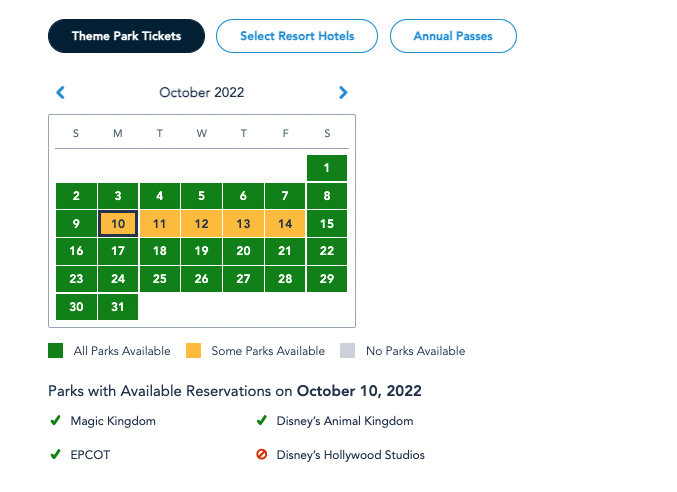This image captures a digital calendar interface, likely viewed on a mobile device or tablet. At the top of the interface are three navigation buttons. The first button, labeled "Theme Park Tickets," is highlighted in black. The adjacent button on the right reads "Select Resort Hotels," and the third button says "Annual Passes." Directly beneath the navigation buttons, the date "October 22nd" is displayed, flanked by blue arrows on both the left and right sides, suggesting functionality to navigate between dates.

Below the date, a monthly calendar is presented, spanning from Sunday to Saturday, with the days of the week represented by their respective initials (S, M, T, W, T, F, S). Most of the individual date squares are highlighted in green, indicating "All Parks Available." However, the dates 10th, 11th, 12th, 13th, and 14th are highlighted in yellow, signifying "Some Parks Available." There are no gray-highlighted dates, which would indicate "No Parks Available."

Further down, the interface explains "Parks with Available Reservations on October 10th, 2022," followed by a checklist: Magic Kingdom, Epcot, and Disney's Animal Kingdom are marked with check signs, denoting availability, whereas Disney's Hollywood Studios has a circled line symbol, indicating no availability for that date.